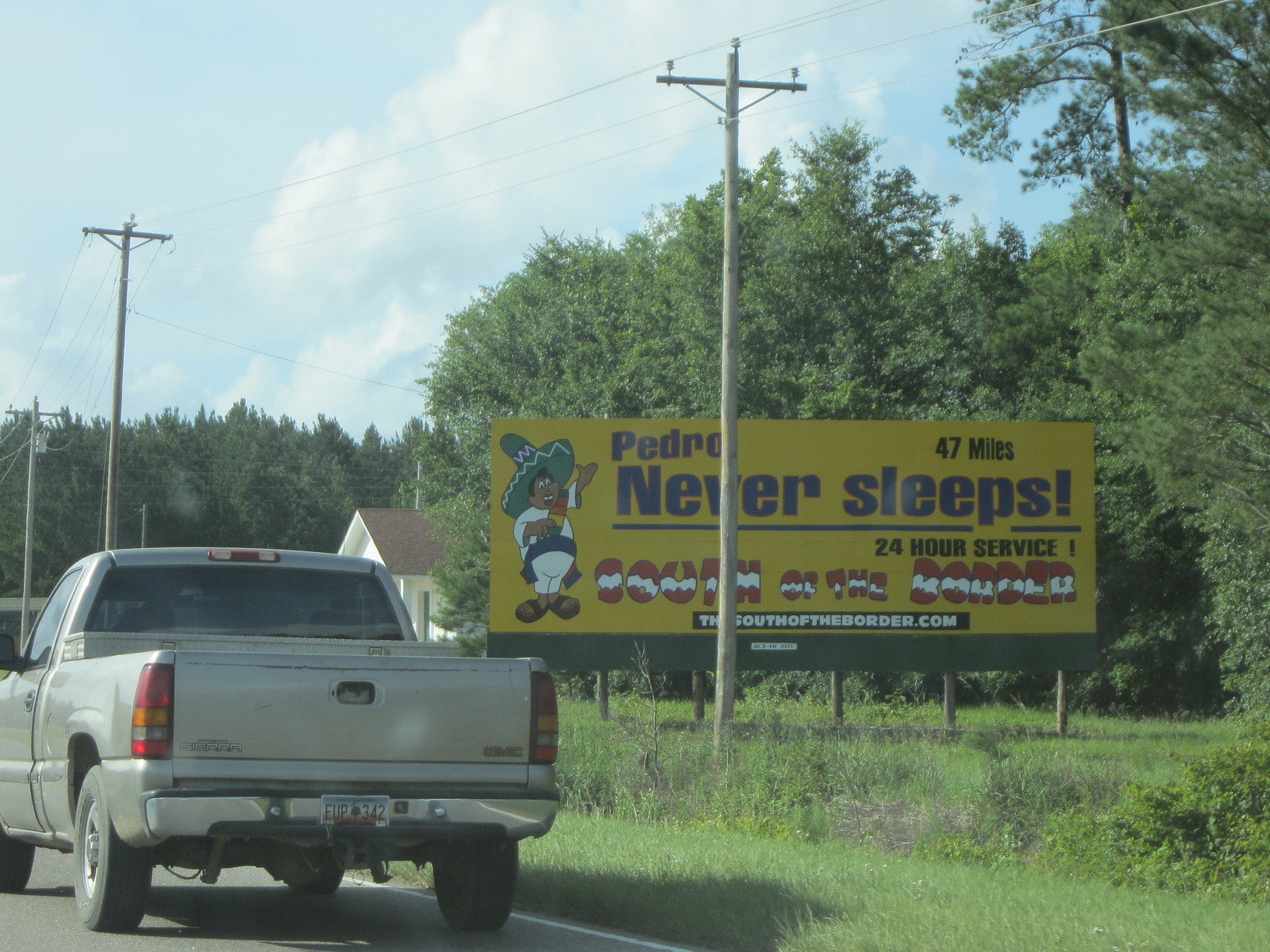In this landscape-format outdoor photograph, a grey or beige GMC truck is seen driving away from the viewer on a paved road, positioned on the left side of the image. The right side of the truck is demarcated by a white boundary line along the edge of the road. Adjacent to the road lies an expansive area of untamed grasslands, which extends roughly 10 feet before transitioning into a mix of weeds and bushes. Beyond this, approximately 50 feet further, the scenery transforms into a forested area.

Dominating the foreground is a large billboard advertisement for "Pedro Never Sleeps," a 24-hour service located 47 miles away. The billboard also features the tagline "South of the Border" with a website URL "thesouthoftheborder.com." The billboard is supported by six wooden posts and is partly obscured by a power line pole. Additionally, a few more power lines stretch across the top left of the image, emerging from above the truck and extending towards the forest line. 

Situated between the power lines, the truck, and the billboard, on the middle left-hand side of the image, a glimpse of a white house with a brown roof is visible. The house appears partially obscured, with only a small section—potentially a window or a doorway—being discernible. Completing the composition, the top of the image reveals a clear blue sky adorned with scattered white clouds, providing a serene backdrop to the rural scene.